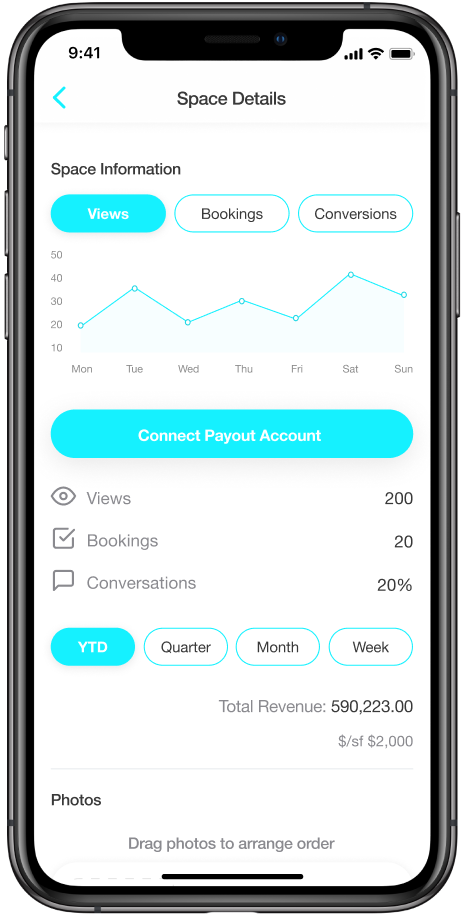In this detailed image, we observe a mobile phone of a dark gray to black color, featuring a sleek rectangular shape with rounded corners. On the left-hand side of the device, there are three buttons: a smaller button near the top followed by two equal-sized buttons placed one beneath the other. Additionally, on the right-hand side, there is a single, large button positioned somewhat close to the top.

The mobile phone's screen displays an app with a white background. At the top of the app interface, we see the title "Space Details," followed by sections labeled "Space Information," "Views," "Bookings," and "Conversions." The "Views" section is currently selected, revealing a line graph below. This graph is plotted with the vertical axis marked at intervals of 10, up to 50, presumably representing the number of views.

The horizontal axis displays the days of the week: Monday through Sunday. The line graph provides a visual representation of the views across these days. Below the line graph, there is a prominent blue button labeled "Connect Payout Count."

Further down, we see a summary with metrics: "Views: 200," "Bookings: 20," and "Conversions: 20%." A section below this summary offers a time frame selection, displaying options for "Year to Date," "Quarter," "Month," and "Week," with "Year to Date" currently chosen. Finally, the total revenue for the selected period is shown as "$590,223."